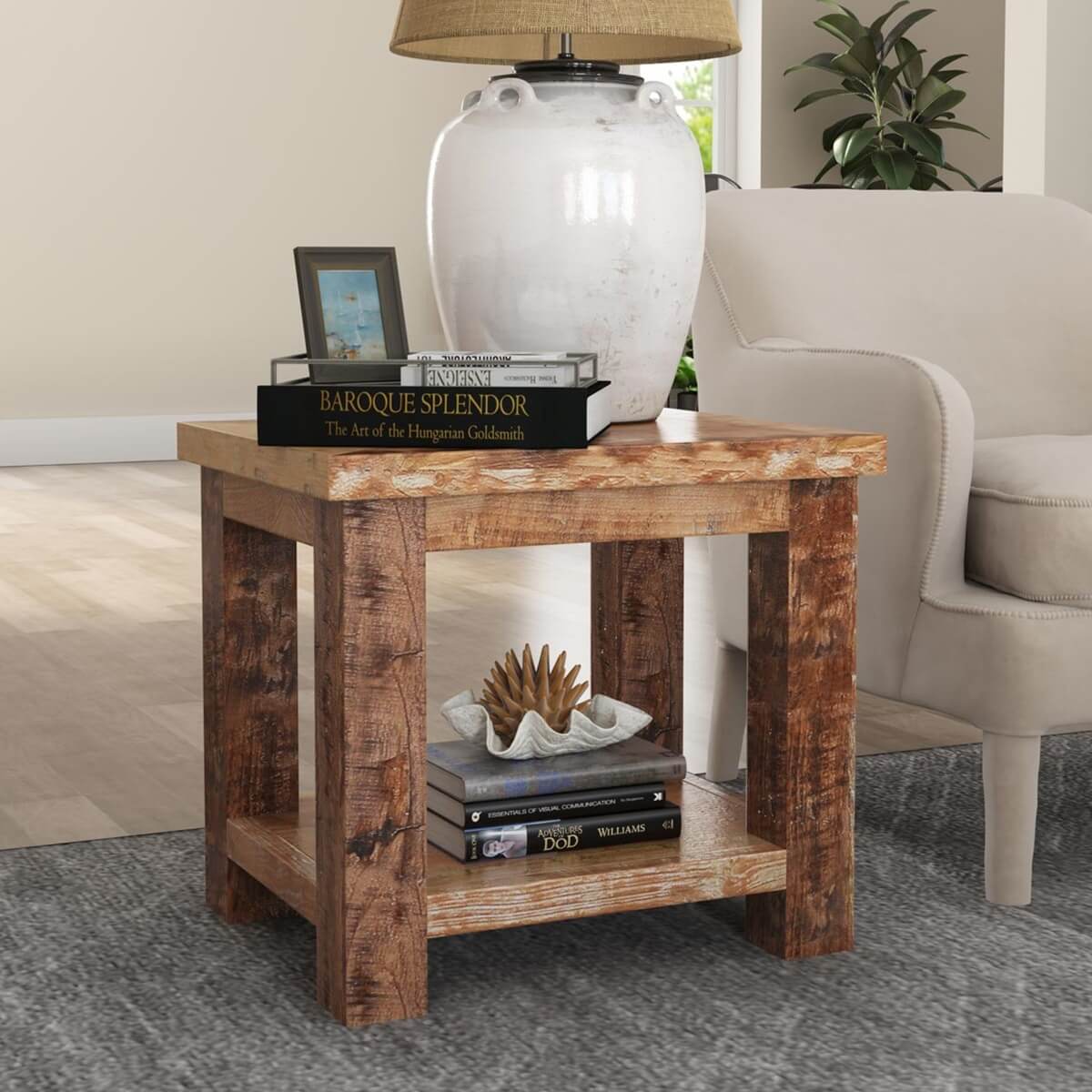The indoor photograph captures a meticulously curated living room scene centering around a wooden end table with a light brown finish and thick legs. This end table, polished and well-designed, exudes an air of sophistication, fitting for a home decor magazine spread. The primary tabletop features a white ceramic lamp with a tan lampshade, casting a gentle light on a black book titled "Baroque Splendor: The Art of the Hungarian Goldsmith," which is inscribed in gold writing. Beside the book, there's a gray picture frame showcasing what appears to be a beach scene, though the details of the photo are indistinct. Additionally, two white books with black writing, their titles illegible, rest on the table. The lower shelf of the end table is adorned with three more black books, all with white lettering, the bottommost bearing the author's surname, "Williams." Atop these books, a ceramic seashell sits elegantly, accompanied by a spiny, possibly wooden, object. Surrounding the end table, a gray fabric chair shares space with a dark gray rug, set against a backdrop of light wood flooring, white walls, and a vibrant green houseplant in the corner, all illuminated by clear, bright lighting.